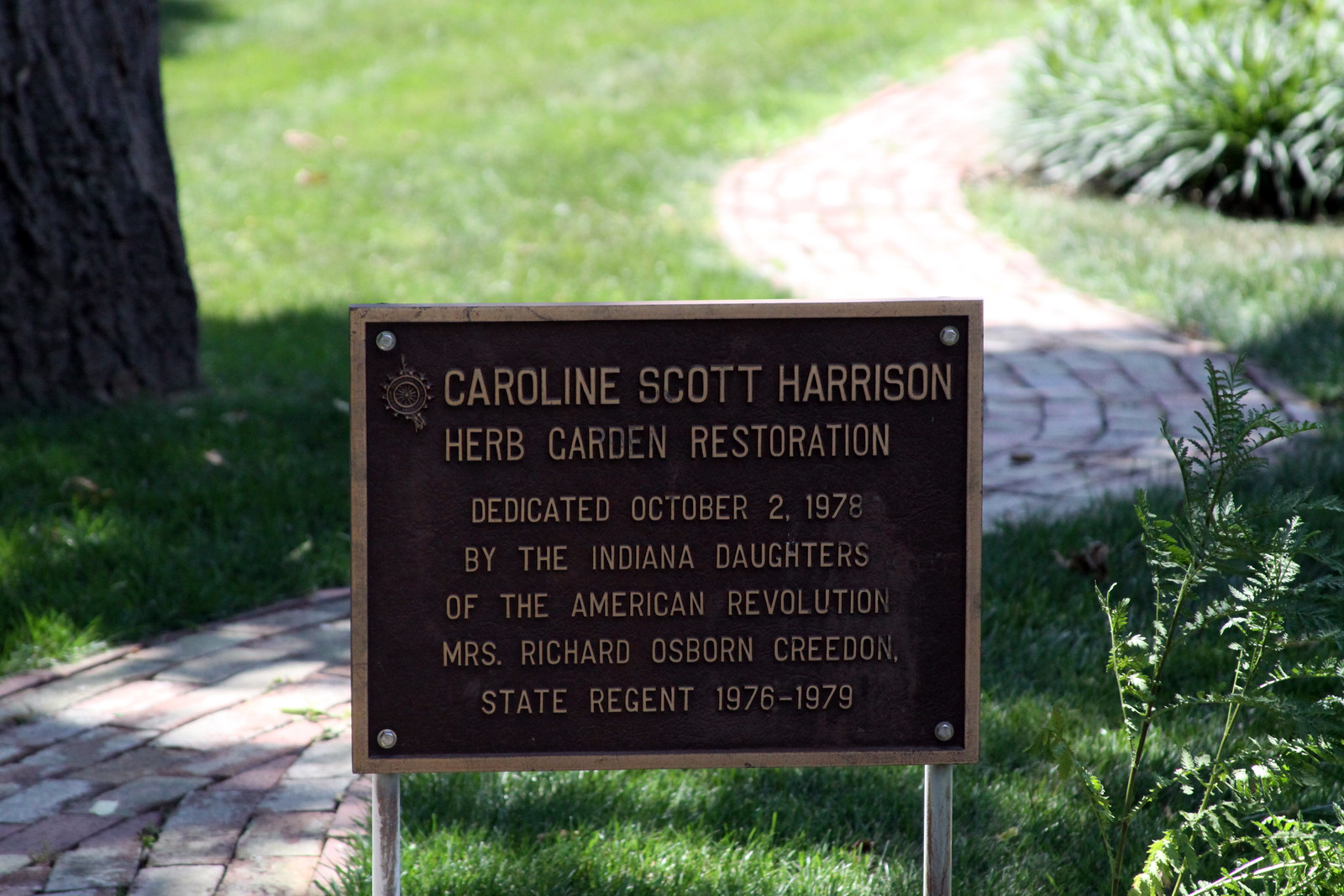The photograph features a brown sign with a gold rim, mounted on two wooden legs embedded in the grass. The sign reads "Caroline Scott Harrison Herb Garden Restoration, dedicated October 2nd, 1978 by the Indiana Daughters of the American Revolution. Mrs. Richard Osborne Creeden, State Regent, 1976-1979." The sign is prominently positioned in the center of the image, with a stone brick pathway winding next to it. The pathway is composed of variously colored bricks, predominantly white, and is flanked by grass on both sides. To the left of the sign, the trunk of a tree is visible, while to the right, bushes populate the scene. The overall setting appears to be an outdoor garden area, illuminated by daylight, reflecting hues of brown, green, red, pink, and tan.